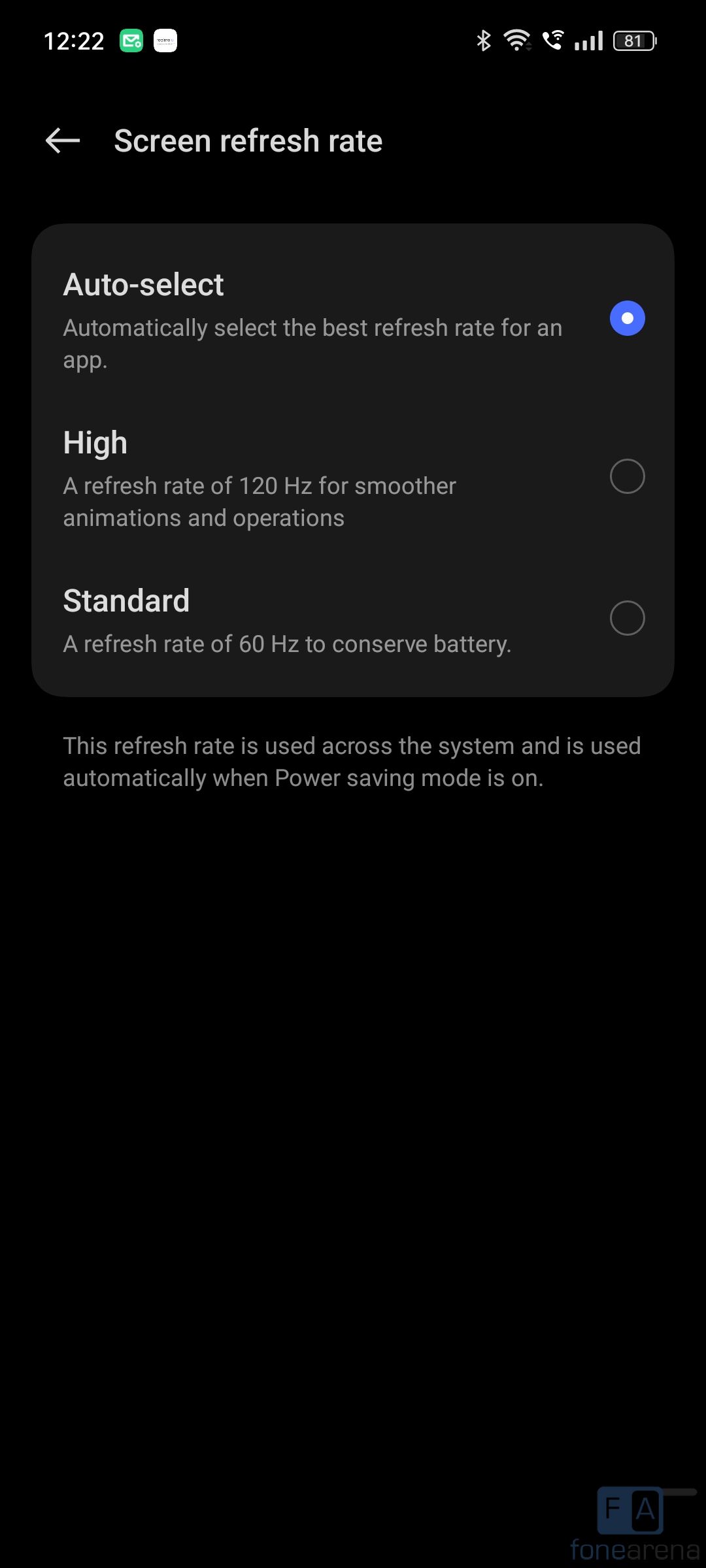This screenshot from a smartphone, identifiable by the time "12:22" displayed at the top left and the battery icon showing "81" at the top right, appears to capture a settings page in dark mode due to the black background. The title "Screen Refresh Rate" heads the page, indicating that the user is adjusting the refresh rate settings on their device. 

Three options are listed: 
1. **Auto Select**: Currently selected, as evidenced by the blue dot next to it, this option automatically chooses the optimal refresh rate for each app.
2. **High**: Offers a refresh rate of 120Hz for smoother animations and operations.
3. **Standard**: Provides a refresh rate of 60Hz, aimed at conserving battery life.

At the bottom, it mentions that this refresh rate applies system-wide and is automatically enabled when power-saving mode is activated.